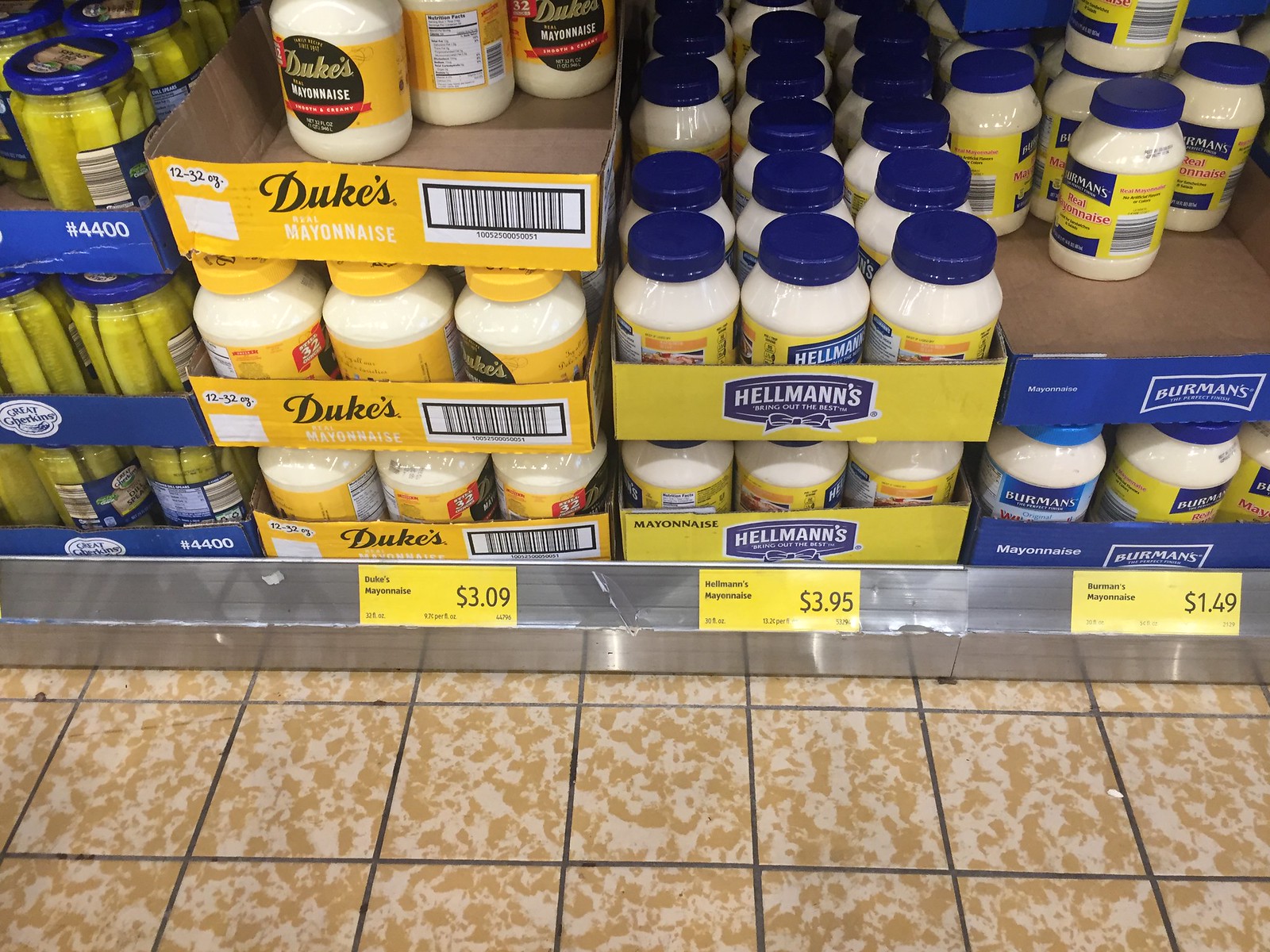This photograph appears to have been taken at Sam's Club, as indicated by the recognizable labels. On display are various condiments, with the left side of the image showcasing three flats of Claussen pickles. Each jar of pickles is uniformly arranged, bearing the distinctive Claussen branding. To the right side of the photo, there are three rows of mayonnaise flats neatly stacked. The brands and prices of the mayonnaise are clearly visible: Duke's mayonnaise is marked at $3.09, featuring a distinctive yellow label and matching yellow lid; Hellmann's mayonnaise is priced at $3.95, identifiable by its yellow label, blue logo, and blue lid; and Berman's mayonnaise, the least expensive at $1.49, has packaging with a yellow and blue label and a blue lid. The organized display and the labels' details make the distinctions between the brands explicit for potential buyers.